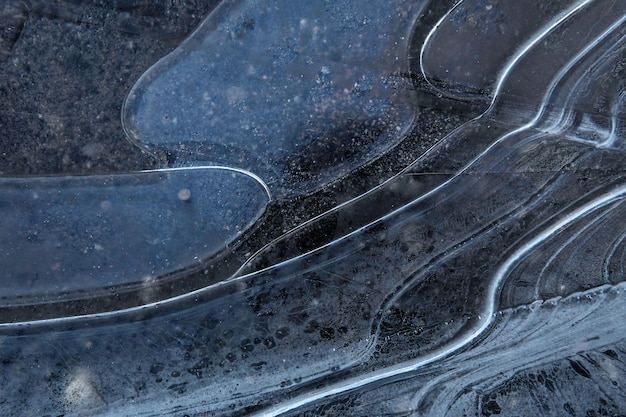This rectangular photograph is a close-up view of what appears to be a partially frozen surface, likely a sidewalk or stone pavers. The image is dominated by shades of gray, black, and white, giving the impression of a textured, stony background. On top of this surface, there's a blend of shiny, round patches and swirling patterns, suggesting the presence of partially frozen liquid, possibly with soapy water that has left behind soap suds. The ice has seemingly undergone stress, with some areas showing cracks and a cloudy appearance, while the liquid areas exhibit a thick, viscous quality. Bubbles are visible beneath the ice, indicating repeated freezing and melting cycles. The overall effect is a mix of smooth and rough textures, creating a dynamic interplay of light and dark across the photograph.